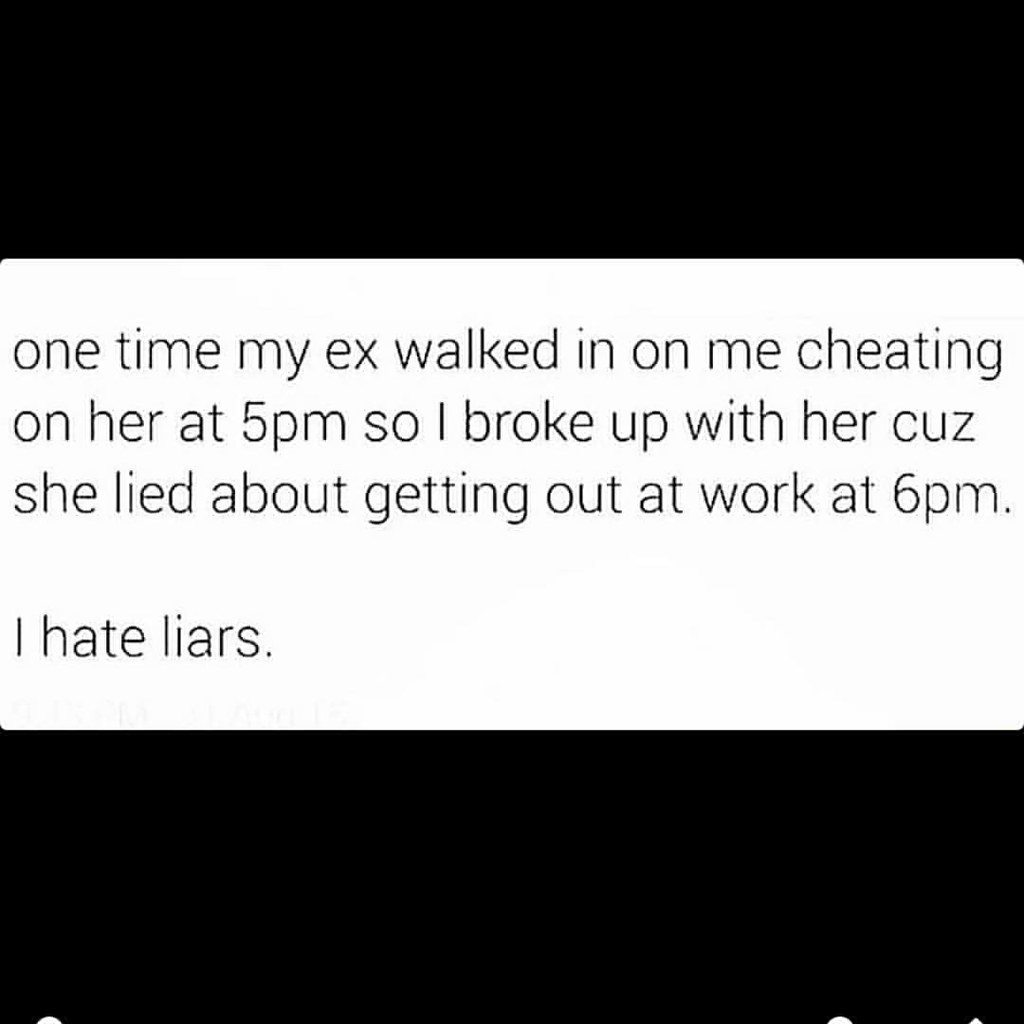This image is a large, perfectly square format featuring prominent black and white sections. The top and bottom portions of the image are solid black bars, creating a stark contrast with the white section sandwiched between them. Within the middle white section, there is a block of left-aligned, all-lowercase black text. The text reads as follows:

"one time my ex walked in on me cheating on her at 5 p.m. so I broke up with her cuz she lied about getting out at work at 6 p.m.

i hate liars."

This text is arranged in three lines, with a space before the final line "i hate liars." Additionally, towards the bottom of the image, near the left side, there is a small arch of white space within the bottom black bar. On the bottom right corner of the image, within the black bar, a triangular white section is also noticeable. The overall composition conveys a narrative of an individual's disdain for deception, illustrated through a minimalist and bold visual design.